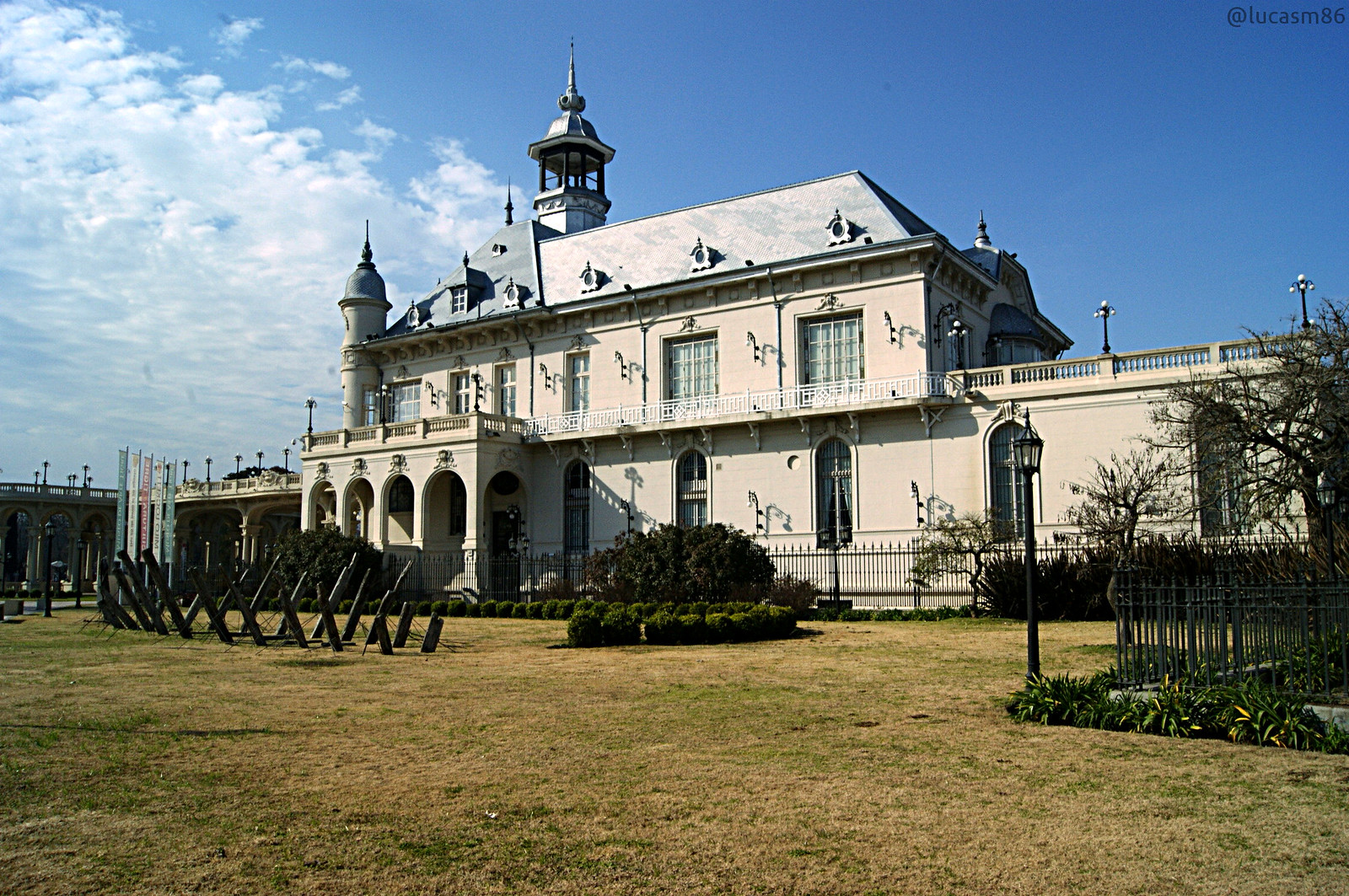This photograph captures a large, cream-colored, European-style estate that seems to hail from the 18th or 19th century, characterized by a tall, peaked roof and distinctive architectural elements. The building, potentially three to four stories tall, features a high-pitched gray roof adorned with small windows and culminates in a prominent tower with a pointed top, likely a cupola or bell tower, on the left side. The front of the estate showcases a stone portico with four arches, supported by columns, that extends to a balcony with a balustrade above it, complete with tall, rounded-top windows on the ground floor and square windows with white frames on the second floor. An additional wide balcony with a railing projects from the right side of the building. In the immediate vicinity, the yard is noticeable for its short, thin grass that appears mostly brown and dry, interspersed with organized shrubs, and metal stakes of uncertain purpose, possibly historical artifacts. A small tree stands on the right, enclosed by a railing. The scene is bathed in sunlight, under a bright blue sky partially filled with puffy white clouds.